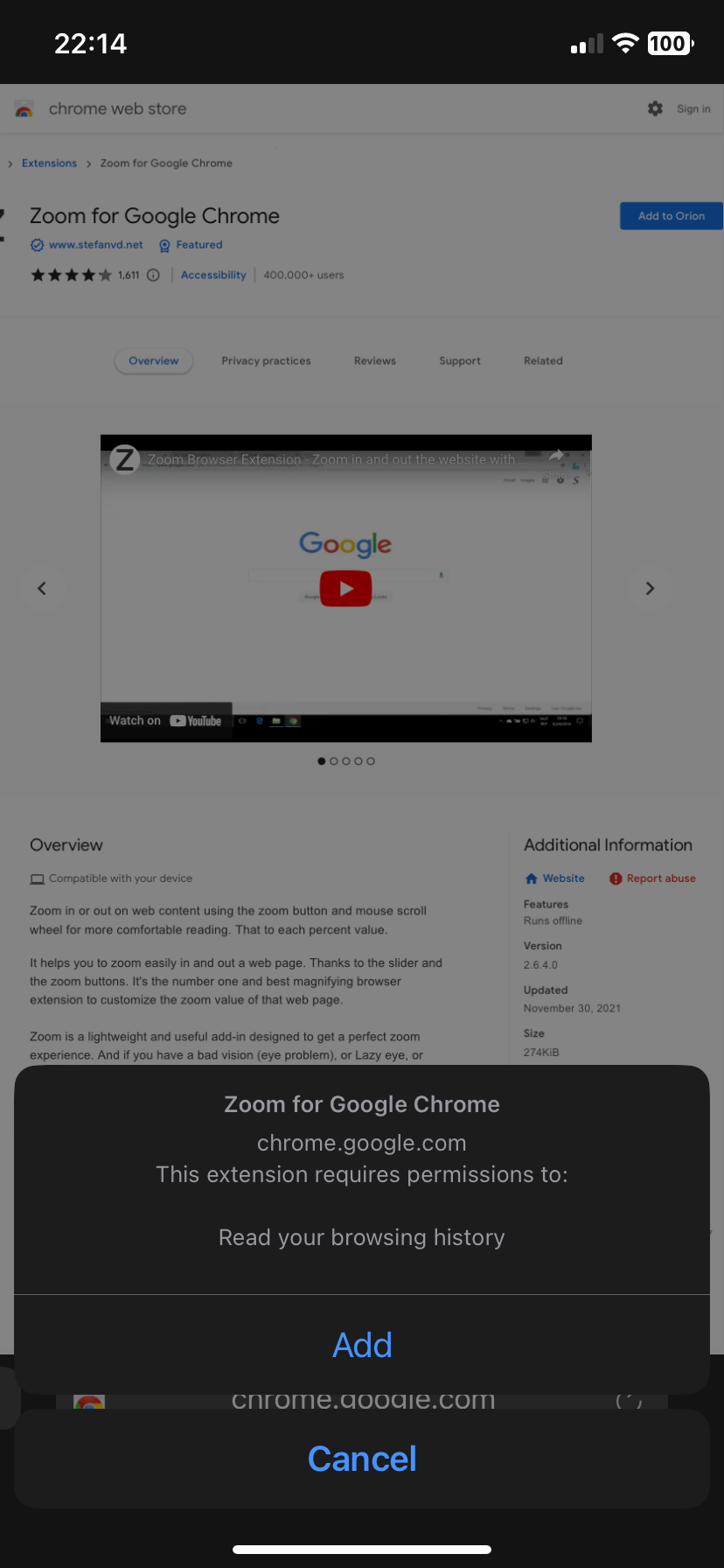The image depicts a screenshot of a browser window showcasing the Chrome Web Store. The top of the screen is black, displaying the time "22:14" and a full battery icon in white. 

Below the black header, the middle section is gray and slightly foggy, featuring small print that reads "Chrome Web Store." An icon of the Google Chrome logo is on the left, and a "Sign in" option is on the right.

Centered on the screen is the listing for "Zoom for Google Chrome" with accompanying small text above and below it. There is a five-star rating visible, and a blue button on the right side. The first of five smaller buttons is blue and highlighted.

Further down, there is a miniature screen with black areas at the top and bottom, including a small black circle with the letter "Z" inside and the word "Google." Adjacent to this is a red square with a white arrow, paired with an arrow pointing left, and text below it.

At the bottom of the image, there is a black box outlining details for "Zoom for Google Chrome" from the URL "chrome.google.com." It mentions that the extension requires permission to read browsing history, accompanied by two blue buttons labeled "Add" and "Cancel."